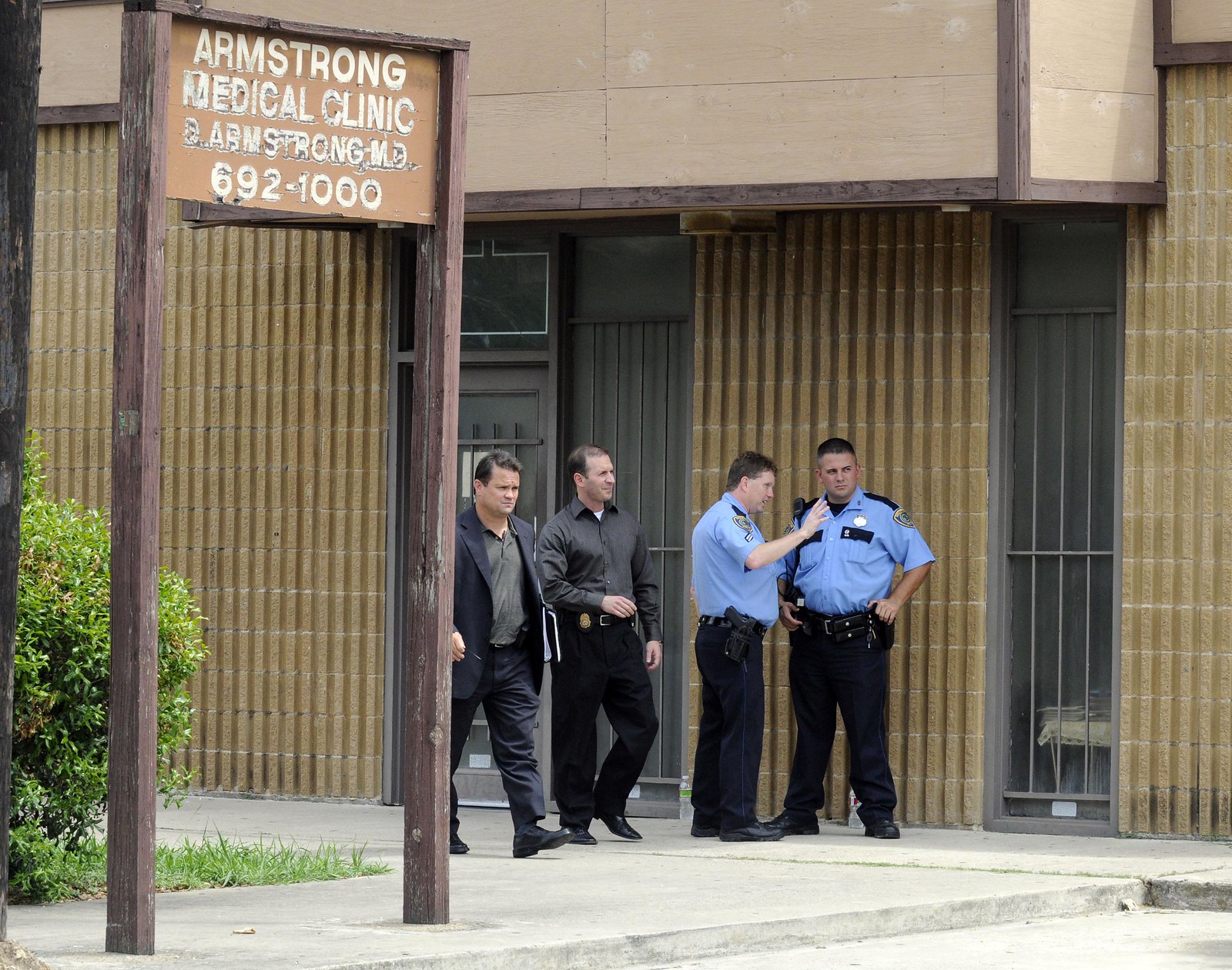In the photo, four men are positioned in front of a building with barred windows, identified by a sign on the left that reads "Armstrong Medical Clinic, D. Armstrong, M.D. 692-1000." Two men, possibly plainclothes officers or detectives, are walking together on the sidewalk. The first man is wearing a sports coat, blue pants, and a gray shirt, while the second man is dressed in a button-down long-sleeve shirt and blue pants; both have badges at their waist. Standing off to the side, engaged in conversation, are two uniformed police officers. They are dressed in light blue short-sleeved shirts with black striped pockets, matched with dark pants, black shoes, and holstered guns. Insignias adorn their sleeves, and radios are clipped to their right shoulders. The setting includes a tree and some bushes near the sign, clearly marking the scene as outside during daytime.